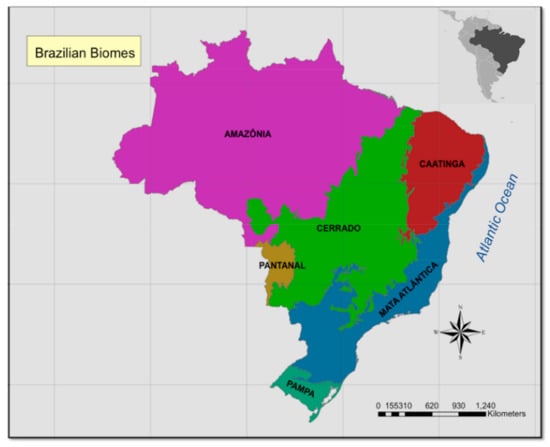The image is a gray, rectangular map of Brazil, slightly wider than it is tall, featuring a detailed illustration of the country's biomes. At the top left corner, a yellow rectangular border encloses the title "Brazilian Biomes." The map highlights the six distinct biomes of Brazil—Amazonia, Pantanal, Cerrado, Caatinga, Mata Atlântica, and Pampa—in various bright colors. The Atlantic Ocean is labeled on the right edge of the map. In the bottom right corner, a scale indicates distances ranging from 0 to 1240 kilometers. Above the scale is a compass showing the directions north, south, east, and west. The map is enclosed by a darker gray border on all sides except the top, and it features a subtle grid-like background.